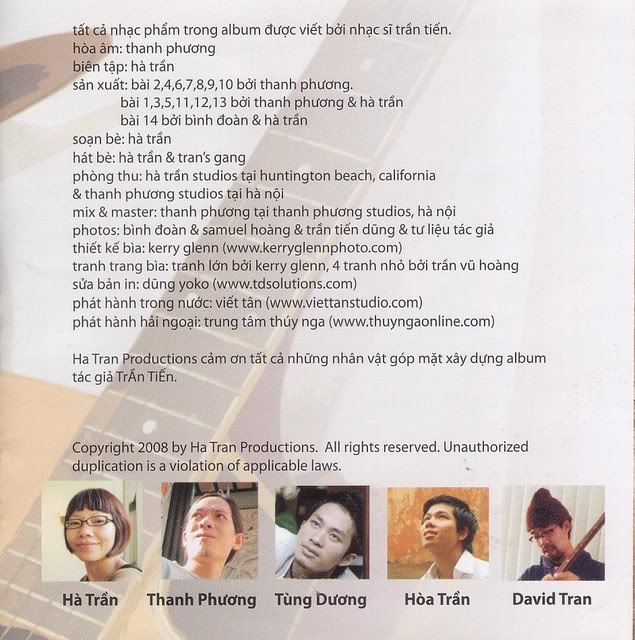This is a detailed poster showcasing the lyrics to a Vietnamese song set against a faded gray background. Dominating the design is a graphic of an acoustic guitar, its light brown body starting from the lower left corner and extending diagonally upward to the right center. The font used for the text is black, standing out sharply against the muted backdrop.

At the top left, paragraphs written in Vietnamese provide detailed information about the album's creation. The text indicates song titles and credits in structured lines. The album is credited to Doak Viet Voa with arrangements by musician Tran Thien Hoa and sound engineering by Thanh Phuong. Production credits include Hoa Tram Studios in Huntington Beach, California, and Thanh Phuong Studios in Hanoi, Viet Nam. Mastering is done by Van Phuong at Thanh Phuong Studios. Contributing photographers and designers listed include Samuel Wong, Trang Tien, and Kerry Glenn. The website links and contact details of the involved studios and people are also provided.

Beneath the text, aligned in a horizontal sequence, are five square headshots of various contributing artists:
1. **Hoa Tran** – A young woman with glasses and short chin-length hair.
2. **Thanh Phuong** – A man looking upward to the upper left.
3. **Tung Duong** – A younger man also looking upward.
4. **Hoa Tran** – Another appearance of the young woman with an orange background.
5. **David Tran** – An Asian man wearing a cap and appearing to play a guitar-like instrument.

At the bottom of the poster, standard copyright information reads: "Copyright 2008 by H.A. Tran Productions, all rights reserved. Unauthorized duplication is a violation of applicable laws."

Overall, this visually appealing poster serves as both a tribute to and a detailed documentation of the collaborative effort behind the Vietnamese album.